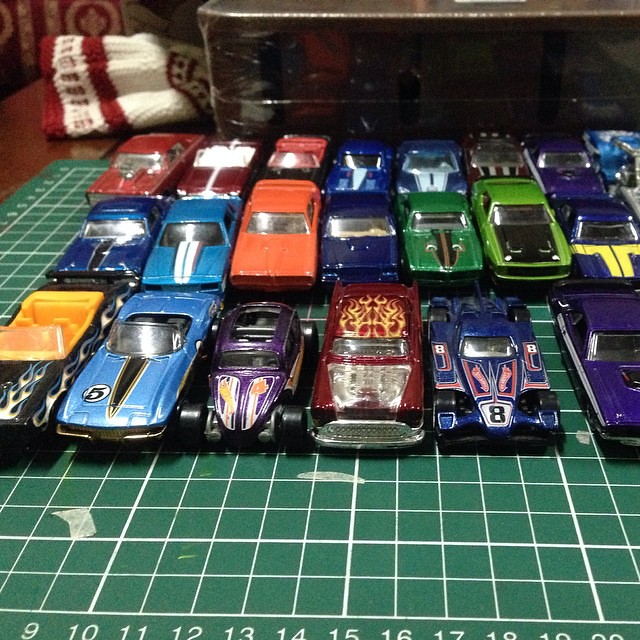This detailed photograph captures an arrangement of 20 meticulously placed die-cast matchbox cars on a green crafting measurement mat, characterized by its white grid lines and numbered increments from 9 to 20 along the bottom edge, though the numbers become less visible beyond 13. The cars are organized into three neat rows, showcasing a variety of colors and styles, including blue, maroon, black, orange, red, green, light blue, purple, and burgundy. Highlights among these vehicles include vintage models, race cars with prominent numbers, and a couple of convertibles. 

The die-cast cars, each approximately 2.5 inches wide and 6 inches long, feature intricate designs such as flames, racing stripes, and number decals. Notable cars include a blue race car with the number 8, a black convertible with orange accents, and a light blue car with a distinctive gold and white triangle stripe. 

In the background, a dark brown wooden table holds the scene, accompanied by a small, metal drawer unit with black drawers just behind the lined mat. Additionally, a red and white crocheted winter hat with lettering around its rim is casually placed on the table in the upper left of the image, adding a touch of warmth to the meticulously staged collection of toy cars.